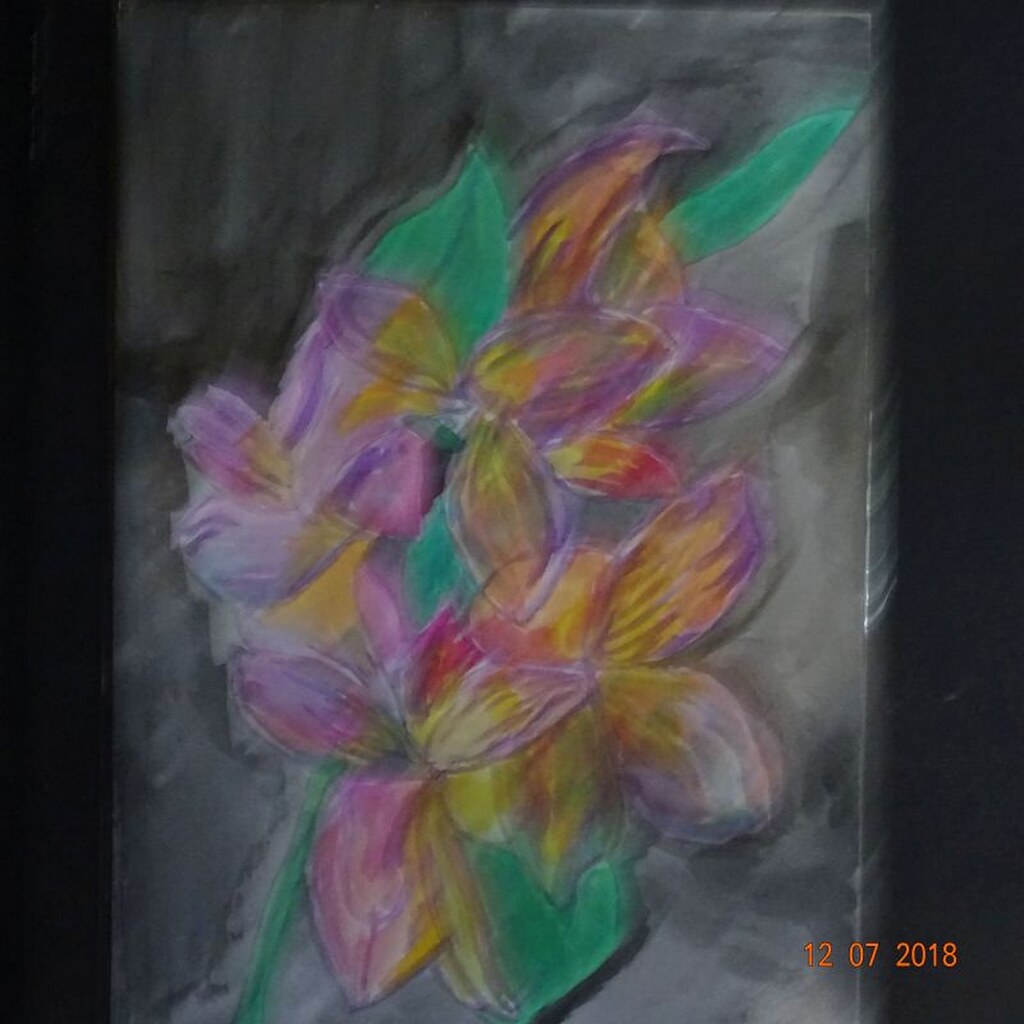This image, captured with a digital camera on December 7, 2018, showcases an amateur artwork set against a background of varying shades of gray and black. The photograph, though blurry, reveals hand-painted or hand-drawn flowers adorned with a mix of vibrant pinks, purples, yellows, and oranges. Complemented by lush green leaves, the floral arrangement elegantly extends from the bottom left to the top right of the frame. Despite the blur, the rich and colorful details of the flowers create a visually captivating contrast against the muted background.